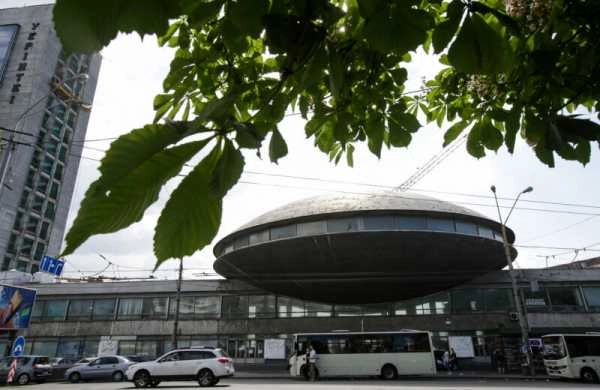This image captures a bustling terminal in an Asian country, framed artfully by the leafy branches of a tree in the foreground. The central feature of the terminal is a distinctive UFO-shaped structure perched atop a long, rectangular, two-story building that spans the width of the image. This terminal serves as a hub for travelers, evidenced by the multiple white buses, cars, and SUVs parked and moving around the entrance. Adjacent to the terminal on the left side of the photo stands a tall, grey building with a multitude of windows and vertical black lettering, possibly spelling out "Y-E-P-I-N-T-E-I." Street signs, telephone lines, and lampposts contribute to the busy atmosphere. The overall scene exudes a sense of constant movement and travel, with an overcast sky completing the urban tableau.